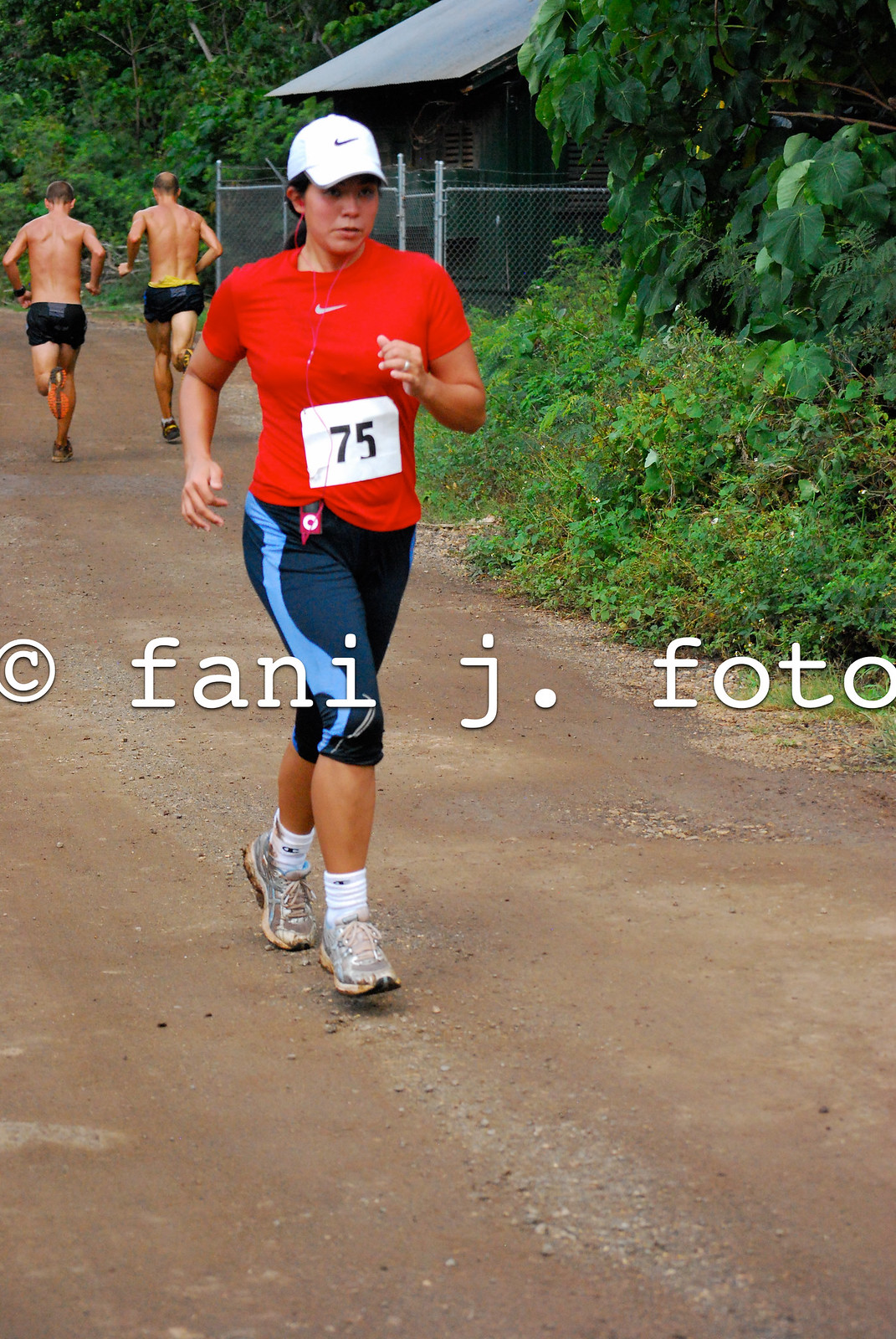In a vertically rectangular, medium-lit photo taken outdoors on a dirt road with a lush, rainforest-like landscape, an Asian woman is the central focus. She is sprinting towards the camera, slightly looking to her right. She sports a red Nike shirt adorned with the iconic swoosh logo, and her race bib features the number 75. Her outfit is completed with dark blue athletic pants that have a light blue stripe down the side, white ankle-high socks, and gray running shoes that display a tan-orange hue. On her head, she wears a white Nike cap, her brown hair tied back in a ponytail. Behind her, two shirtless men in black shorts are running in the opposite direction, their backs turned to the camera. To the upper right of the frame, a large shrubbery is visible, while the upper left corner shows part of a cabin-style building with a chain-link fence. A watermark reading "Fanny J. Photo" runs through the center of the image.